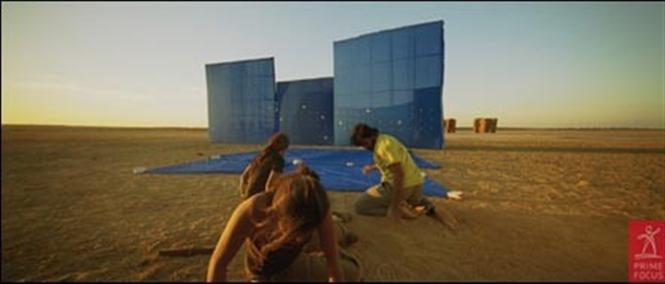In this detailed and surreal desert landscape, the scene is set against a flat, sandy expanse stretching to the horizon, with colors of light blue and yellow painting the sky, indicative of either a sunrise or sunset. In the foreground, three individuals are engaged in what appears to be a meticulous search or setup process on the ground. The group consists of a man in a yellow shirt and two women, all positioned on their knees and facing away from the camera. One woman is more hunched over as if closely inspecting or working on something in the sand.

Central to the image is a large blue tarp, secured with rocks to prevent it from blowing away. This tarp stretches over the sandy terrain and behind it stand three tall, flat, blue structures resembling reflective solar panels or glass walls. Further back, indistinct light brown objects emerge from the sand, possibly art pieces or buildings, but they remain just out of focus.

In the lower right-hand corner of the image, there is a distinctive red box logo depicting a stick figure with outstretched arms and the words "Prime Focus" inscribed underneath. This logo hints at the purposeful activity taking place within this meticulously detailed and otherworldly desert setting.